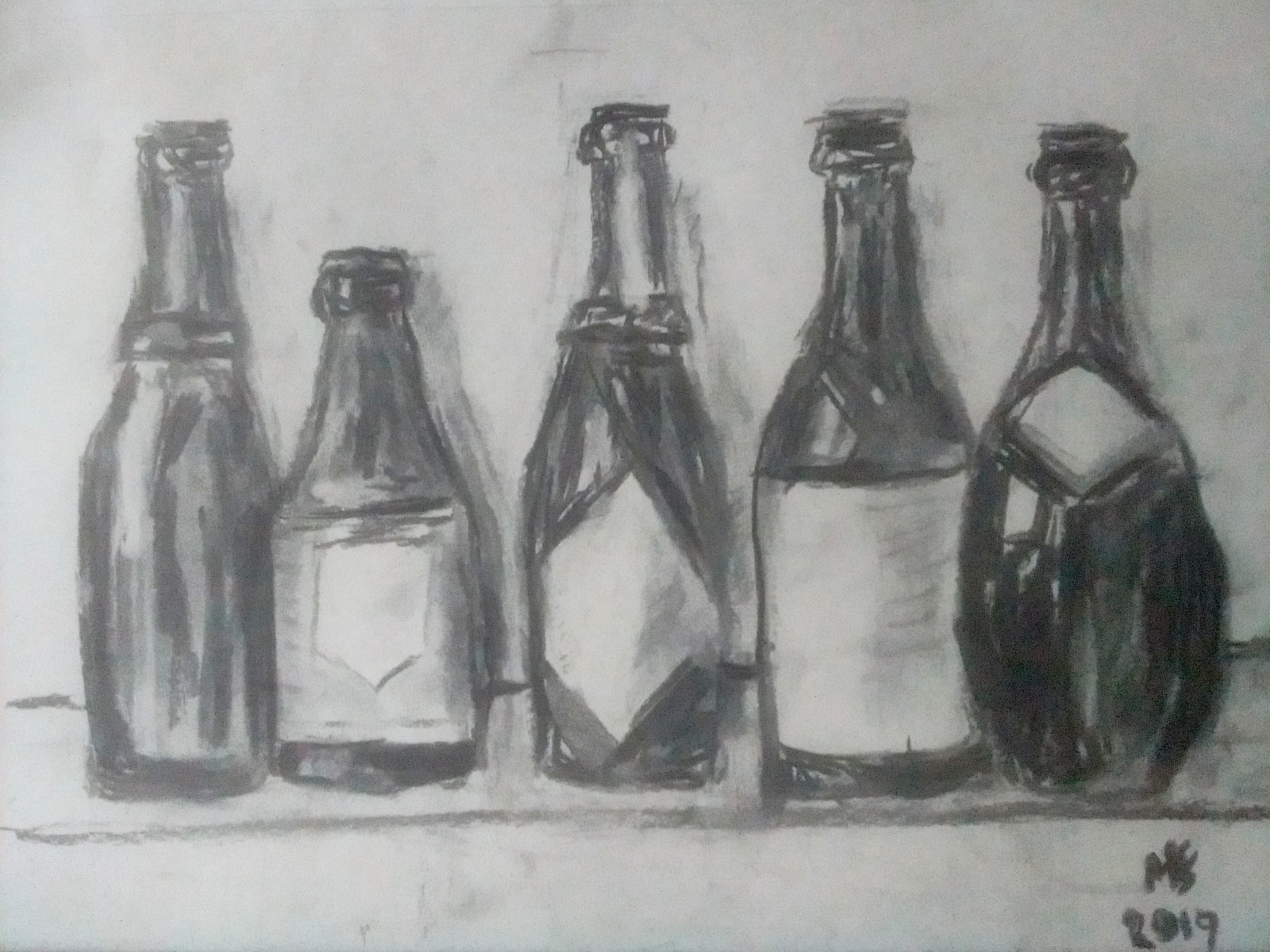This captivating sketch features five meticulously drawn bottles, each distinct in appearance and color. Despite the initial sketchy feel, the detailing is impressive, with each bottle clearly outlined to convey its unique shape. The bottles appear to be empty, as they lack definitive lids. The colors vary, ranging from transparent hues on the left to a darker bottle on the right. The darkest bottle, located on the far right, stands out with its elongated oval body and a diamond-shaped embellishment on its shoulder. The artist's signature, "M.F. 2017," is elegantly placed in the bottom right-hand corner, adding a personalized touch to this intriguing and aesthetically pleasing piece.